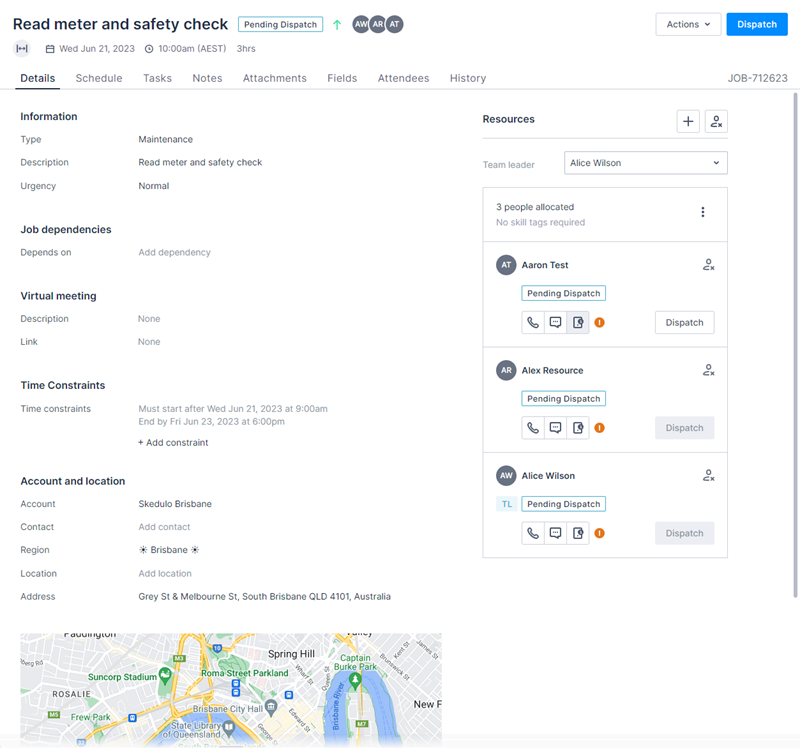The image depicts a detailed interface related to a task management system, focused on "Read Reader and Safety Check." Set against a white background, there is a prominent square button labeled "Pending Dispatch" next to the words "Read Reader" and "Safety Check." Additionally, three small black circles, each containing the letters A-W, A-R, and A-T in white text, are visible. A green upward-facing arrow button is present, indicating possibly a status or navigation button.

The interface was captured on Wednesday, June 21, 2023, at 10:00 AM (AEST) spanning a duration of three hours. Different sections are highlighted for details, schedule, tasks, notes, attachments, fields, attendees, and history.

Under the "Information" section, it shows the type, description, and urgency of the task:
- Type: Matency
- Read Reader and Safety Check
- Urgency: Normal

In the "Job Dependency" section, it indicates "depends on" with an option to add dependencies. No virtual meetings are scheduled, with no descriptions or links provided. Time constraints are outlined as:
- Must start after: Wednesday, June 21, 2023, at 9:00 AM
- End by: Friday, June 23, 2023, at 6:00 PM

The "Account and Location" section specifies:
- Location: Skidooleo, Brisbane
- Address: Gray Street at Melbourne Street, South Brisbane, QLD 4101, Australia
- Map: Displayed at the bottom

The "Resources" section lists Alice Wilson as the team leader and three allocated members: Aaron Tess, Alex Resource, and Alice Wilson. Their dispatch statuses indicate 'Pending Dispatch' for all, but Aaron Tess’s button is active, while Alex Resource’s and Alice Wilson’s buttons are grayed out.

At the top of the interface, an "Actions" menu is visible with "Dispatch" highlighted in blue. The task is identified by job number 712623.